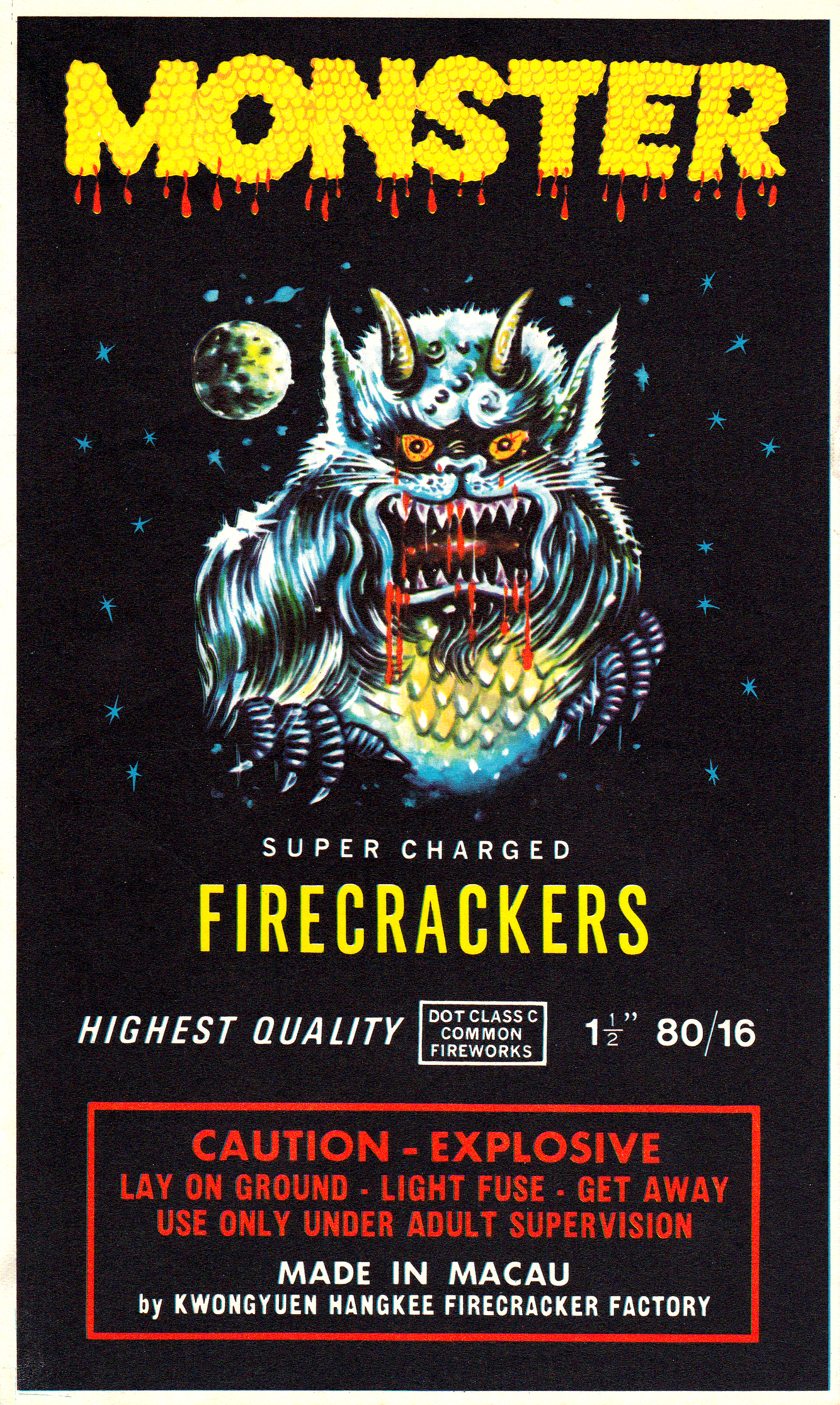The image depicts an intricately designed black poster. At the top, bold yellow text reads "MONSTER," accented with red droplets that resemble blood dripping down the letters, creating a striking and ominous effect. Dominating the center is a large, menacing monster, drawn in an 80s cartoon style. This creature has pointed horns, large ears, yellow bloodshot eyes with black pupils, and sharp white teeth dripping with blood. Its blue fur contrasts with its scaly chest and eagle-like claws. Surrounding the monster is a celestial background with blue stars and planets, and a small moon to the side.

Below the monster, the words "Supercharged Firecrackers" are prominently displayed, with "supercharged" in white letters and "firecrackers" in yellow. Further down, in smaller text, it reads "Highest Quality . Class C Common Fireworks," followed by "1 1/2 inch 80/16." Encased in a red rectangle at the bottom, red text warns: "Caution - Explosive. Lay on ground. Light fuse. Get away. Use only under adult supervision." Beneath this warning, in white letters, it states, "Made in Macau by Kongyang Hanqi Firecracker Factory." The overall design combines vivid imagery with critical safety information, blending an intense visual style with practical details.